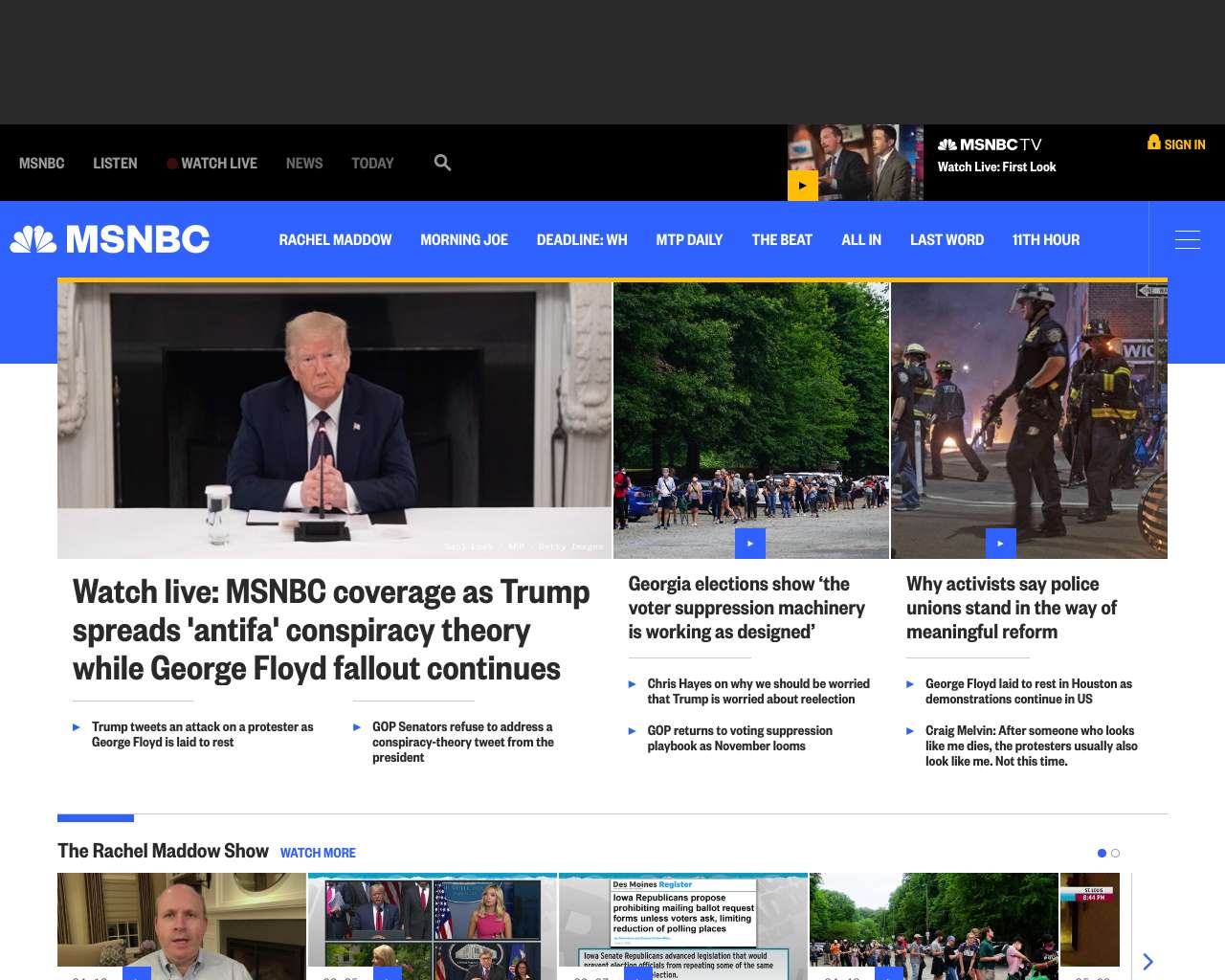The image captures the MSNBC website highlighting several news articles and video features. Dominating the center of the screen is a prominent image of Donald Trump seated behind a desk. The headline accompanying this image reads, "Watch Live: MSNBC Coverage as Trump Spreads Antifa Conspiracy Theory While George Floyd Fallout Continues." Beneath this main story are a few subheadings, providing more context or related content.

To the right of the main article are two related stories focusing on George Floyd. The first article discusses the impact of voter suppression in Georgia elections, with a headline that reads, "Georgia Elections Show the Voter Suppression Machinery is Working as Designed," accompanied by an image and a video. The second article, which also includes a video, is titled, "Why Activists Say Police Unions Stand in the Way of Meaningful Reform."

Additionally, beneath these stories are a series of videos from the Rachel Maddow Show and other MSNBC programs, available for browsing. At the very top panel of the website, just above a blue section, the main MSNBC programs are listed, including Rachel Maddow, Morning Joe, Deadline: White House, MTP Daily, The Beat, All In, Last Word, and The Eleventh Hour. Above this section, the website offers user navigation options including Watch Live, Listen, News, Today, and a search function.